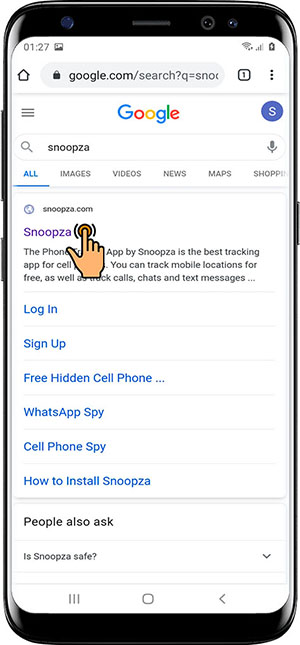The image is a detailed screenshot of a black smartphone, potentially an iPhone or an Android device. The screen shows the glare of sunlight reflecting off its surface. The display is open to Google's search results page, indicating a search query for "Snoop Za."

At the top of the screen, a partial URL is visible: google.com/search?q=Sno. The search results include various tabs such as "Log in," "Sign up," "Free hidden cell phone," "WhatsApp spy," "Cell phone spy," "How to install Snoop Za," and "Is Snoop Za safe." Below these, three lines of text briefly explain the functionality of the Snoop Za service, accompanied by a small image resembling a finger pointing to the right.

Three icons are located at the bottom of the screen, with a blue "S" indicating a logged-in profile. The device displays the time as 1:27 PM and shows a full battery. Additional common Google search tabs like "All," "Images," "Videos," "News," "Maps," and "Shopping" are visible at the top of the search results.

The overall scene conveys the subject's current engagement with a search query and the various informational elements related to Snoop Za on a well-charged mobile device in sunlight.